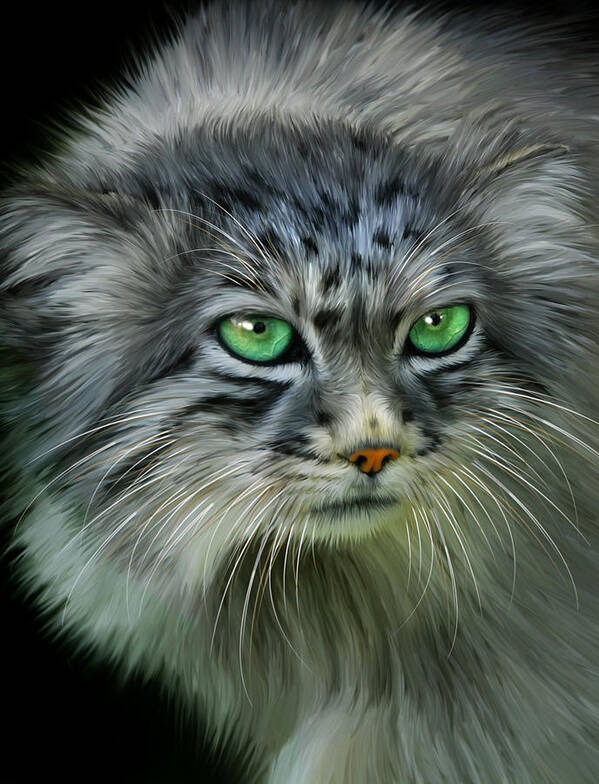This detailed digital illustration depicts a Pallas's cat, or manul, with features that closely resemble those of a house cat, yet distinctively wild. The Pallas's cat boasts long, dense fur in light gray, white, and black hues, giving it a majestic, fluffy appearance akin to having a mane. Its face is broad with rounded ears set low on the sides of its head, accentuating its unique look with exquisite ice-green eyes. The cat's pupils are notably round, a rare sight, adding to the mesmerizing allure of its gaze. Its nose carries a pinkish-orange tint, contrasted by plentiful white whiskers that further highlight its expressive features. Black spots are also discernible on its forehead. The entire illustration, set against a simple black background, captures this small wildcat in stunning detail, giving the impression of a realistic, though digitally created, close-up image within a rectangular frame.